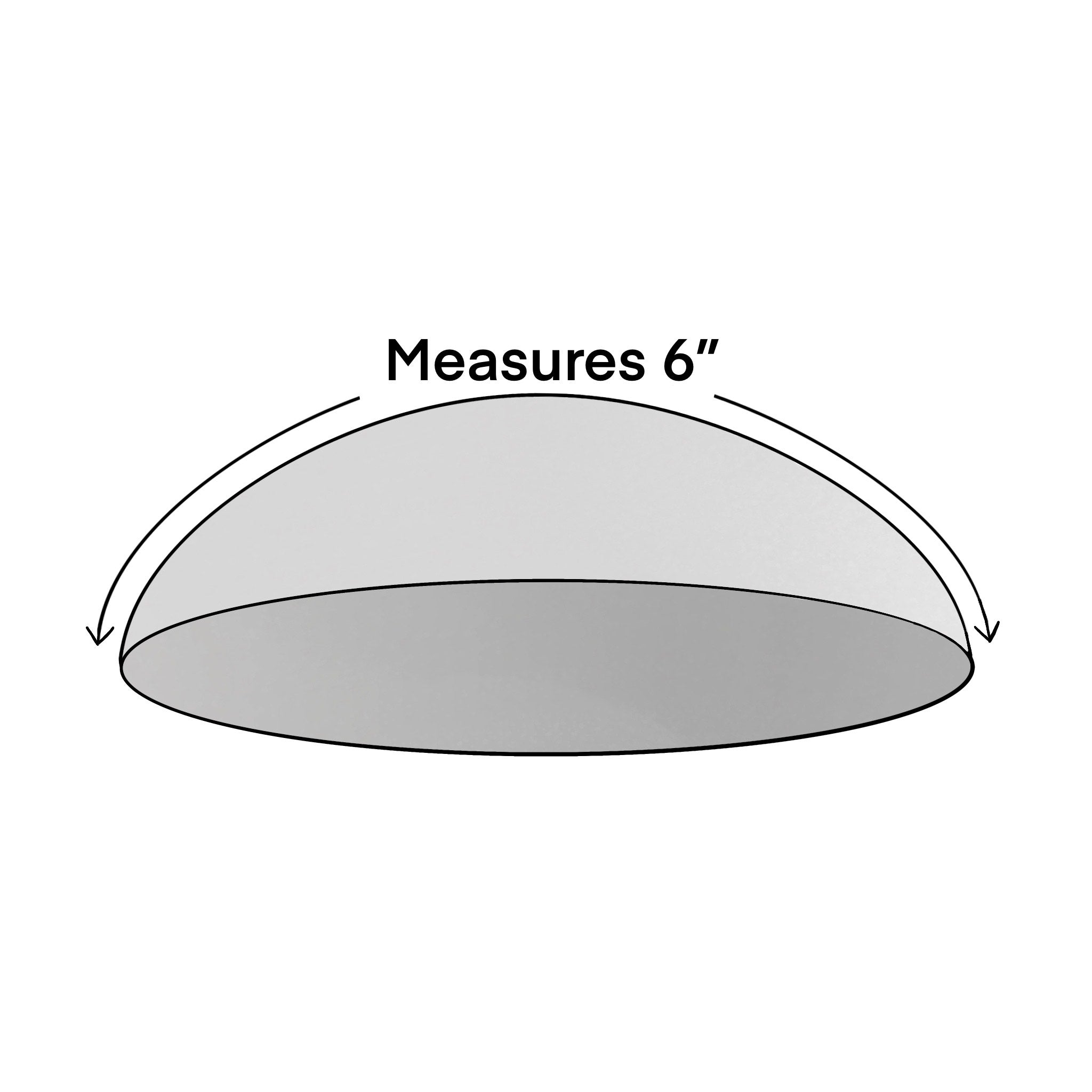The image is a detailed illustration of a gray, dome-shaped object on a white background. The dome appears three-dimensional, giving a realistic feel with a lighter gray shade on the top half and a darker gray at the bottom. In the center of the image, there is a black line, suggesting some form of division or emphasis. At the very top of the dome, there is black text reading "Measures 6 inches," indicating the dome's size. Flanking the dome, two black arrows curve downwards from either side, each pointing towards the base of the dome. The dome's shape, with its flat bottom and curved sides, is depicted clearly and gives an impression of being somewhat see-through. There are no additional objects or details inside the dome or around it, making it a straightforward, focused graphic representation.